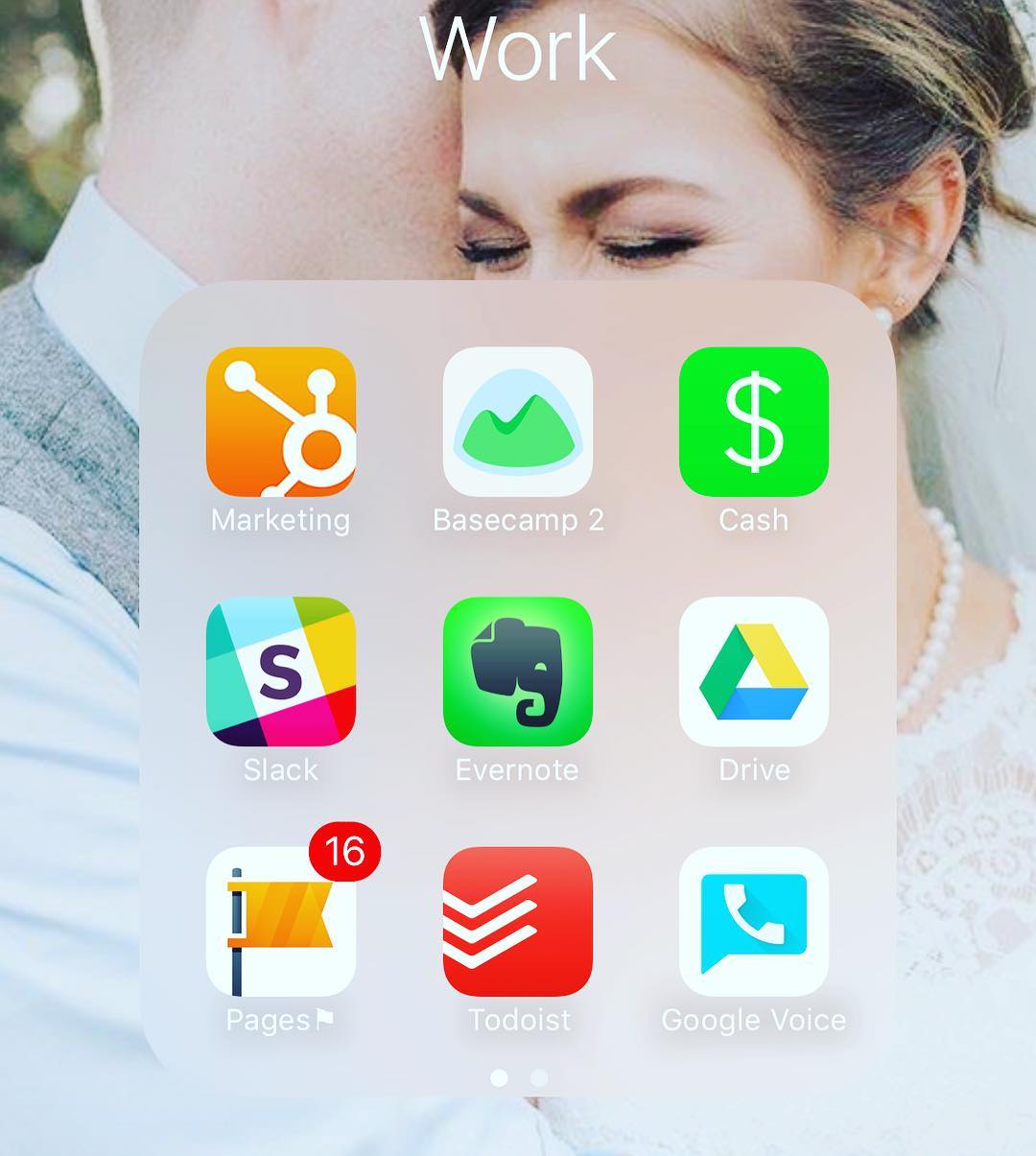This is a screenshot of someone's cell phone home screen, featuring a backdrop of a wedding photo with a bride and groom. The bride's face is partially visible, facing the viewer, but everything below her eyes is obscured by a gray rectangle displaying various app icons. At the top, the word "Work" appears in a thin white font. 

The groom, standing next to and embracing the bride, has his face turned to the side. Only his cheek and a portion of his ear are visible, as the rest of his head is cropped out of the image. The bride is adorned in a white dress and a pearl necklace, while the groom sports a powder blue shirt underneath a gray and black tweed vest.

The phone's screen displays three rows and three columns of apps. From top to bottom and left to right, these apps include:
1. A marketing app, represented by an orange square with white graphics.
2. Basecamp, illustrated with a white square and green logo.
3. Cash App, marked by a green square with a white cash symbol.
4. Slack, denoted by a plaid symbol with an "S" in it.
5. Evernote, a green square featuring an elephant silhouette.
6. Google Drive, showing the Google logo.
7. Pages app, identifiable by an orange flag on a flagpole with a red notification showing the number "16."
8. Todoist, a red square with three white check marks.
9. Google Voice, depicted by a white box with a blue speech bubble containing a white phone silhouette.

This combination of personal and professional elements showcases the organization and usage of the device owner’s home screen.